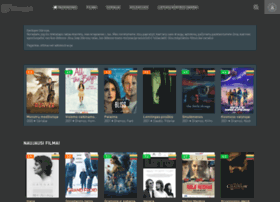This is a screenshot of an application with a dark mode interface, featuring a content selection carousel. The text within the image is somewhat blurred due to the small size. The carousel displays a series of movie posters, allowing users to select a movie based on its cover image. This layout resembles a streaming platform similar to Netflix, where each movie is presented in a tile format. The screenshot shows two rows of movie titles, each accompanied by a brief description beneath the respective posters. Among the visible titles, one features actress Salma Hayek, which stands out as the most recognizable movie in the selection.